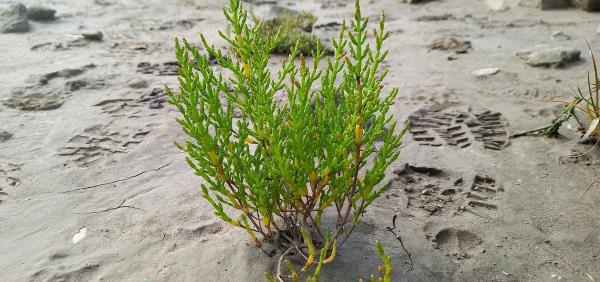The image is a detailed color photograph featuring a desert plant in a dry, cracked soil landscape. This green bush-like plant has thick stems with small, pointy leaves and no flowers. Surrounding the plant are several distinct footprints, likely from a man's shoe, showcasing detailed tread patterns. To the right of the main plant, there's a smaller weed-like plant, and various gray, dry rocks are scattered across the scene. Despite the dry appearance, the soil retains a fine grain texture, hinting at its sandy composition. Additionally, a few shells are interspersed among the rocks, enhancing the rugged, arid setting.